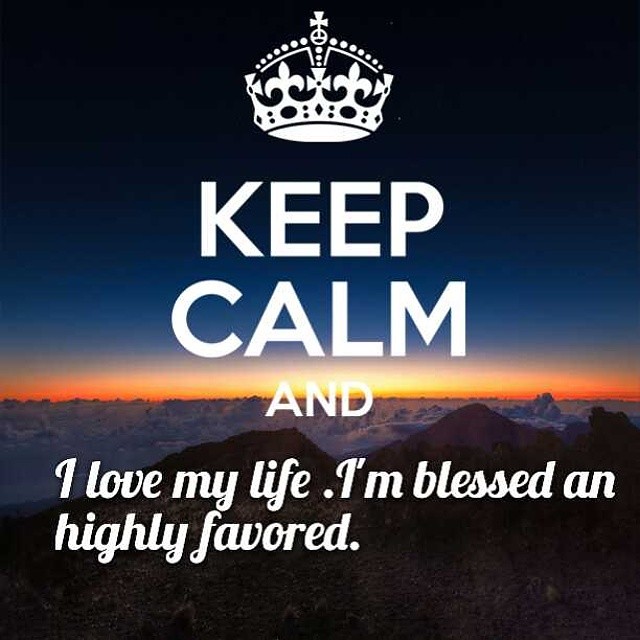The image is a dark advertising poster featuring a prominent white graphic of a king's crown at the top center against a background that transitions from a black sky to a lighter horizon with hues of orange and yellow, suggesting either a sunrise or sunset. Beneath the crown, in large white letters, the text reads "KEEP CALM" followed by "an" (A-N, not A-N-D) in smaller white letters. Below this, in a cursive font, the words "I love my life. I'm blessed and highly favored." are inscribed. In the background, there is a depiction of an ocean with visible water, some rocks, and a beach in the foreground, with mountains in the distance. The overall composition resembles a motivational social media post, blending different font styles and an animated crown, possibly created digitally.